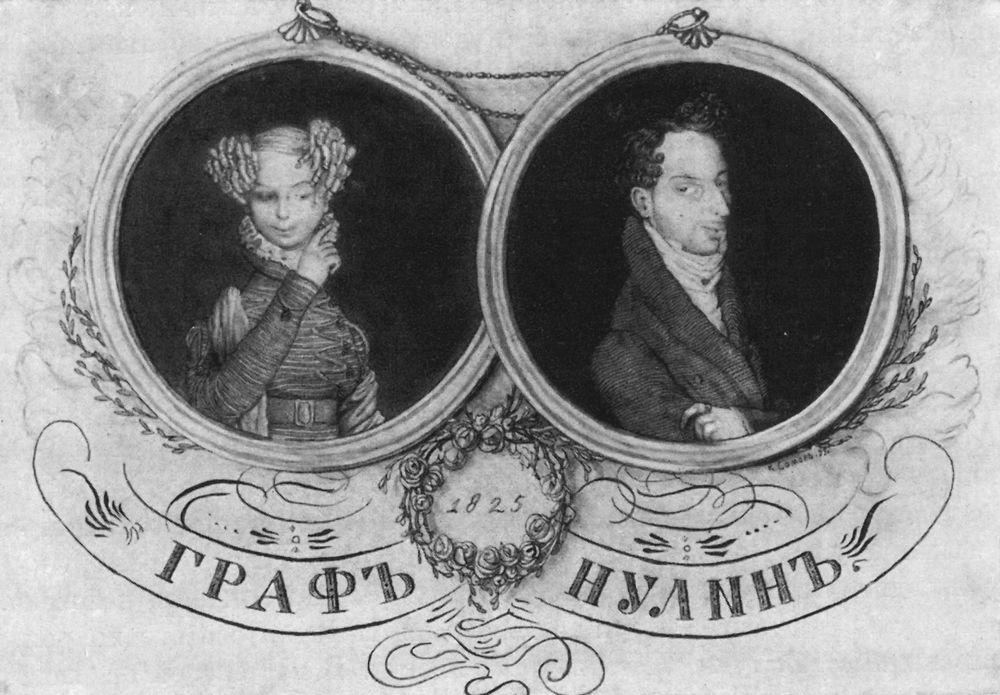This intriguing ink illustration on paper features two vintage-style portraits inside round pendants, connected by a delicate chain. Framed by hand-drawn metallic circles, the central focus includes a woman in the left pendant and a man in the right pendant, both set against completely black backgrounds. The woman, wearing an ornate, frilly-necked dress, has her hair styled in three buns and curls. She points delicately to her ear with her right hand while gazing towards the man with a subtle side glance. The man, dressed in a suave high-neck black overcoat and white shirt, reciprocates the glance, looking back at the woman with a slight turn of his head. His left hand rests across his chest. Below the circles, a black and white drawing of a wreath prominently displays the date 1828. Additional foreign text, resembling Greek letters beneath the woman and Cyrillic beneath the man, is written in a scroll-like manner, adding an extra layer of mystery to the illustration. The entire composition is rendered in detailed black and white pencil drawings against a light gray background.